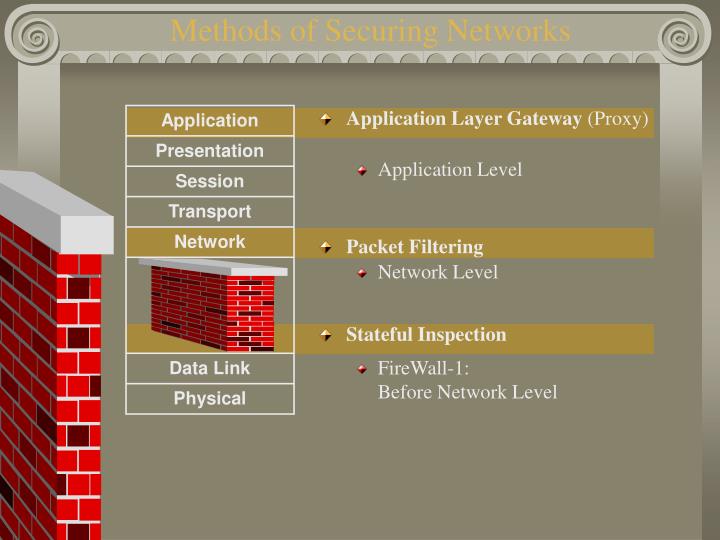The image is an informational page from a computer screen featuring a gray background at the top with the title "Methods of Securing Networks" in yellow letters. Below the title is a table divided into sections, each row representing different network layers. The top row has "Application" highlighted in brown, followed by "Presentation", "Session", "Transport," and another brown-highlighted "Network." Under the network is an image of a red and black brick object with a white top that looks like a chimney, corresponding to the "Data Link" layer, and the last row is labeled "Physical." 

To the right of each layer name, there are gold diamond-shaped bullet points: next to "Application" it says "Application Layer Gateway (Proxy)" with a sub-bullet point "Application Level", and next to "Network" it mentions "Packet Filtering" with a sub-bullet point "Network Level." Next to the brick image, it states "Stateful Inspection" and "Firewall-1: Before Network Level."

On the left side of the screen, from the bottom left corner extending past the middle, is a thin brick column in red and black with a white cap on top, resembling the brick object seen in the table.